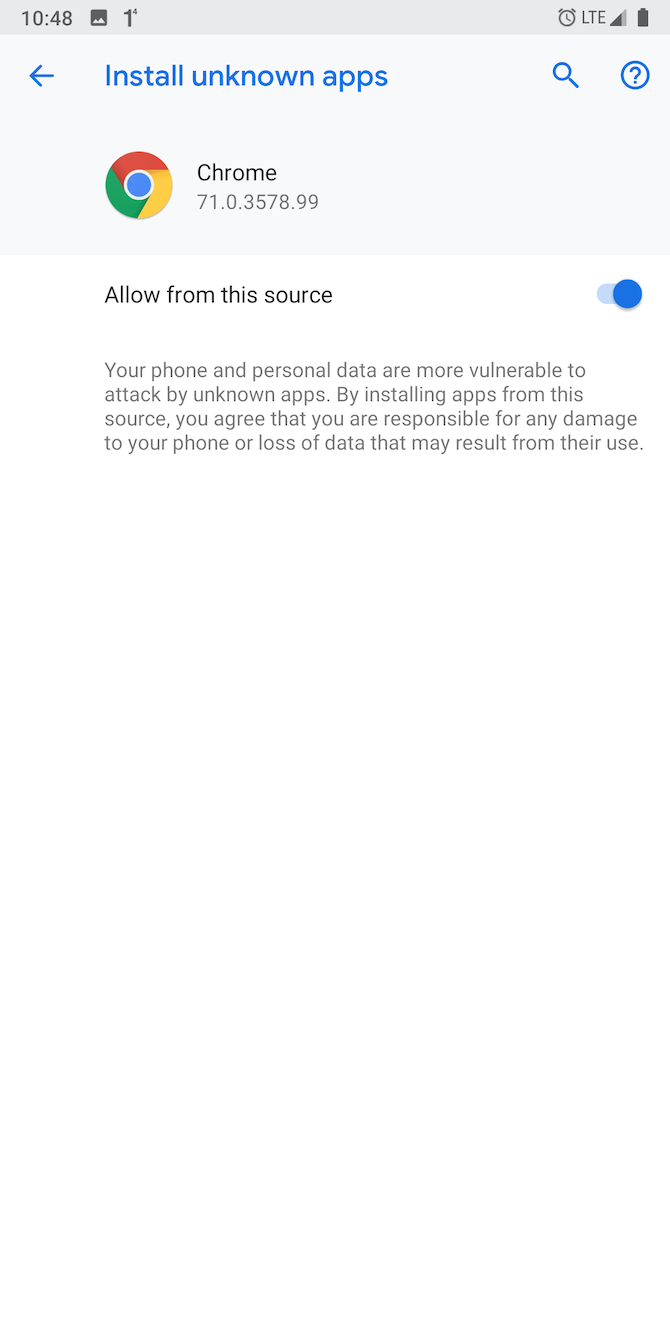Partial screenshot of the 'Install Unknown Apps' section in the settings of an Android mobile device. The image displays the top third of the screen, where you can see the configuration related to the Chrome browser. The Chrome logo, a circle composed of green, blue, yellow, and red colors, is prominently visible, along with the version number 71.03578.99. The option to "Allow from this source" is enabled, indicated by a blue switch, allowing the installation of apps directly from the Chrome browser. This setting is commonly accessed when attempting to install apps from external sources via the Chrome web browser.